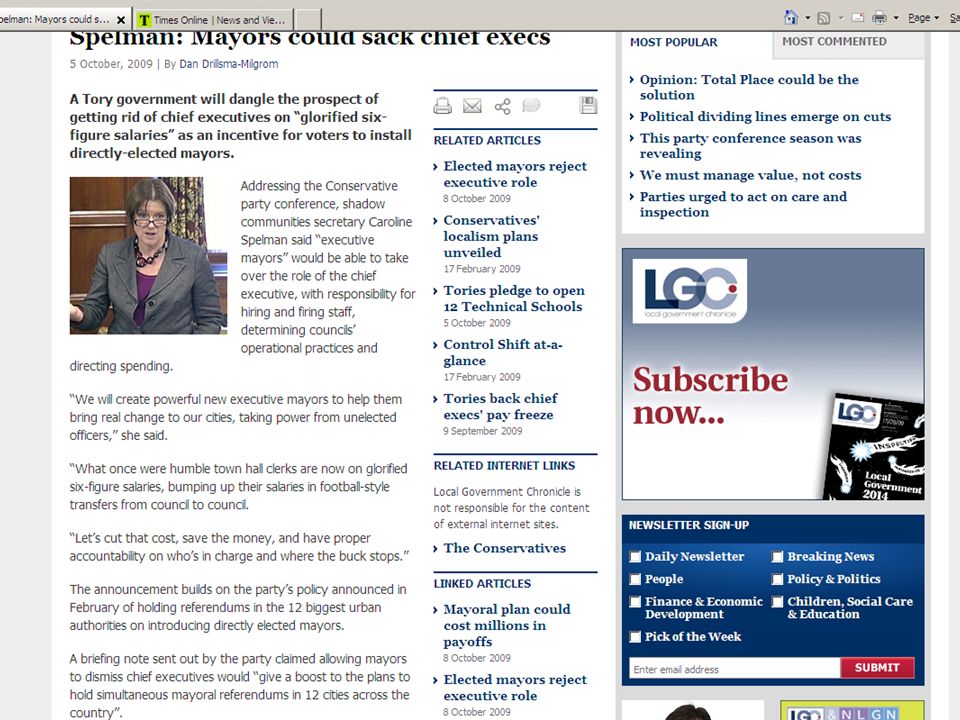A screenshot from an archived 2009 webpage of the Times Online, likely retrieved via the Wayback Machine, depicts an article discussing potential political changes in the UK, specifically focusing on the powers of directly elected mayors. The top navigation bar displays two active tabs: one labeled "Times Online, News and View" and another partially titled "Spellman Mayors could." Accompanying icons for home, RSS feed, email, and print options are visible, indicative of an older web design format.

The main headline reads, "Spellman Mayors could sack chief execs," dated 5 October 2009 by Dan Jilsmilgram. The accompanying subheading reveals that a Tory government is considering offering voters the ability to sack high-earning chief executives as an incentivizing reform measure. Below the headline, there's an image of a woman appearing at what seems to be a referendum meeting, adding visual context to the political discussion.

To the right of the main article, a sidebar features various sections: related articles linked in blue text, a "Most Popular" list with six topics, and a "Most Commented" section. Beneath these, an advertisement for Local Government Chronicle (LGC) urges readers to subscribe, followed by a newsletter signup form at the bottom, all framed within the distinctively retro layout of a 2009 webpage.